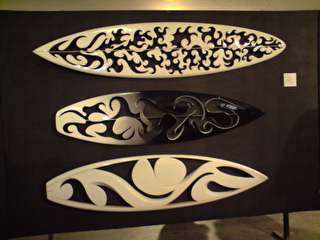The image is a horizontal rectangular photograph showcasing what appears to be a display of intricately designed art pieces. The background features a dark panel with a subtle golden light emanating from thin strips along the top and bottom. Central to the image are three elongated, teardrop-shaped objects that resemble surfboards, stacked vertically with small gaps between them. These objects are detailed with intricate cutout patterns, allowing the dark backdrop to show through. The top piece features leaf-like designs, the middle has wavy patterns, and the bottom one has a sporadic pattern. The objects are likely made of either metal or porcelain, reflecting light in a way that highlights their detailed craftsmanship. To the right of these designs, there is a small golden square, possibly a label or part of the display. The scene gives the impression of a polished and carefully arranged art exhibit, possibly digital or computer-animated due to the precision and clarity of the elements.